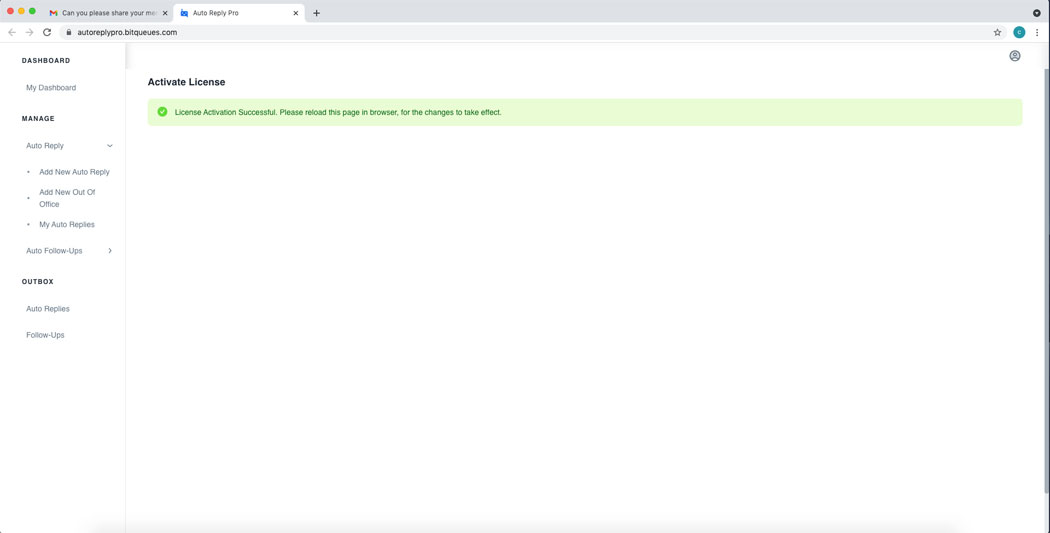The image depicts a web browser window with two tabs open. The active tab displays a webpage belonging to Auto Reply Pro, accessible via the URL autoreplypro.bitqueues.com. On the left side of the page, a vertical navigation menu includes various options: My Dashboard, Manage, Auto Reply, Add New Auto Reply, Add New Out of Office, My Auto Replies, Auto Reply Follow-ups, and Outbox.

The main section of the webpage has a prominent green message that reads "Active License Successful," indicating the active status of the license. Beneath this message, it advises users to reload the page in their browser for the changes to take effect.

The page design features a color palette including red, yellow, green, blue, light green, teal green, gray, white, and black. Despite the colorful elements, the majority of the page is a blank white space, with the focus on the navigation menu and the license activation message.